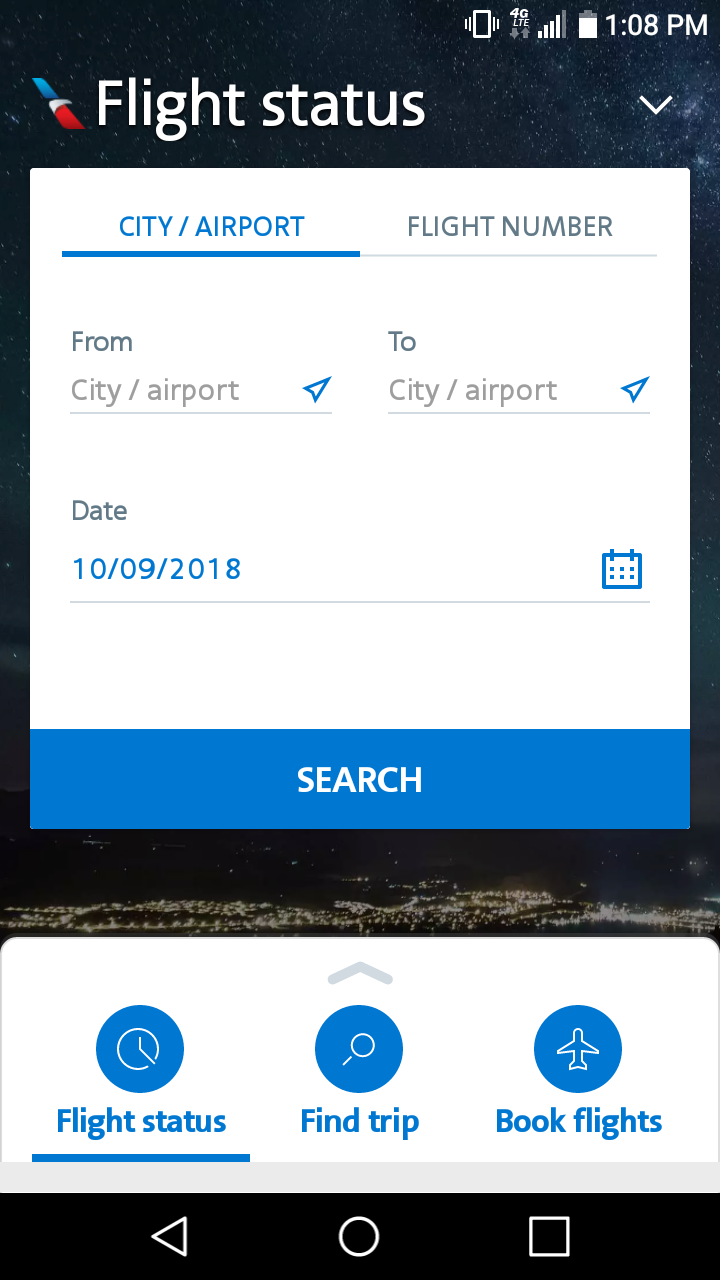The screenshot captures an Android device, identifiable by the characteristic navigation icons—a triangle pointing left, a circle, and a square—located at the bottom. The device is currently on silent mode, as indicated by the status bar at the top, showing a 4G LTE connection with four out of five signal bars and a nearly full battery at 1:08 PM.

The display is focused on a website pertaining to flight information. While the address bar is not visible, the content centers around a flight status search. Dominating the screen is an image of an aircraft's tail, featuring a diagonal design transitioning from blue to white to red, suggesting it could belong to Southwest or American Airlines.

The screen prominently features a "Flight Status" title with a drop-down arrow, under which users are given the option to search by "City/Airport" (currently selected in blue text) or "Flight Number" (displayed in gray text). Beneath this, users are prompted to enter information for either the departure or arrival city/airport, illustrated by an icon of a paper airplane taking off. The date is set to October 9, 2018, with an adjacent calendar icon indicating the option to change the date.

Below this input section is a blue "Search" button in a rectangle with white text. Further down, three additional options are displayed within blue circles: a clock icon labeled "Flight Status," a magnifying glass icon labeled "Find Trip," and a plane icon labeled "Book Flights," suggesting further functionalities that can be expanded upon.

Overall, this screenshot showcases a web interface designed for checking the status of flights, highlighting the necessary tools and fields for users to input and search for flight information.